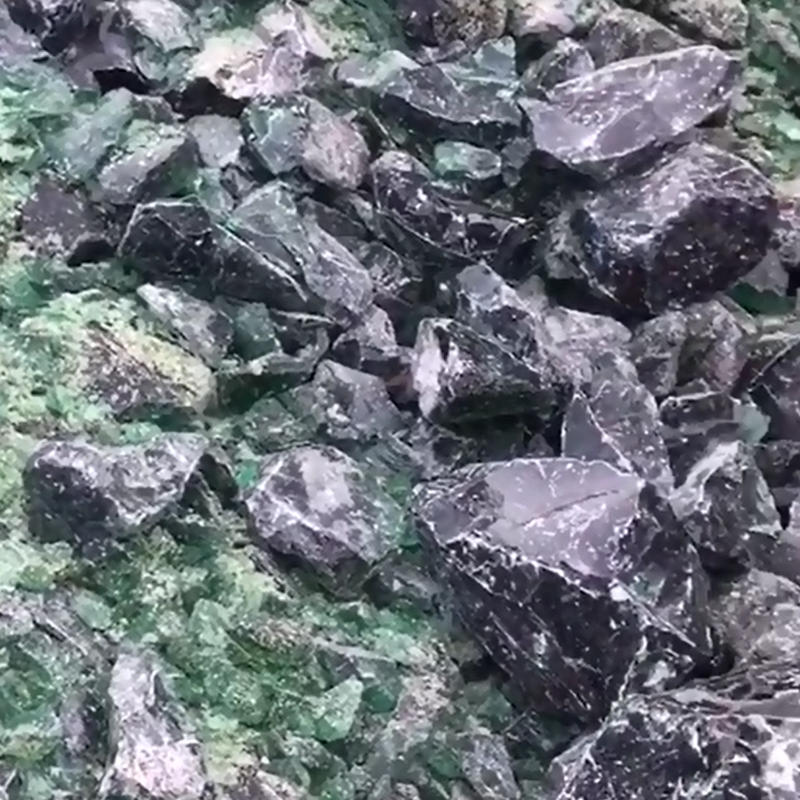This color photograph, presented in a square format, captures a closely-packed array of jagged, unpolished crystal-like rocks scattered across the entire frame. The dominant objects in the image are large black crystals with striking white veins, reminiscent of obsidian or marble. These dark, flat rocks, primarily positioned on the right and upper right side, are complemented by smaller, gravel-like green crystals, which also bear white streaks and splashes. The green stones are mostly positioned on the lower left, extending upward and across the top of the image. This natural and rugged arrangement suggests a setting possibly linked to a mine or a facility for processing minerals. The photograph's realistic, representational style further emphasizes the textural details and variations in color, including shades of black, green, white, gray, and hints of turquoise.